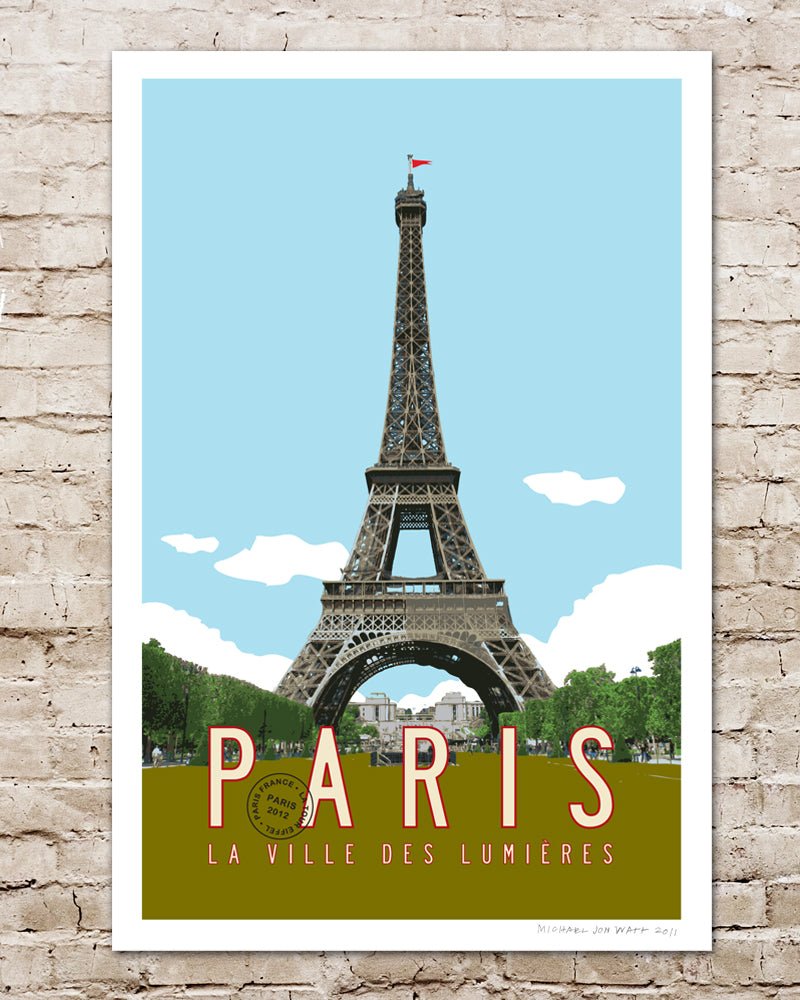The poster of Paris is prominently displayed on a weathered, whitewashed brick wall that features cracks and dings, adding character to the scene. The poster itself is framed by a thick white border, drawing the eye to the vibrant image it encloses. Central to the poster is an artistic depiction of the Eiffel Tower, standing tall against a clear blue sky dotted with three fluffy clouds. The Eiffel Tower, portrayed in a metallic silver color, narrows gracefully towards the top and broadens at the base, descending into four sturdy legs. Flanking the tower's base are rows of lush green trees, leading forward toward the viewer and framing a patch of brown-green grass in the foreground.

Highlighting the cultural prominence of the scene, large white lettering at the bottom of the image reads "Paris," with smaller text beneath it stating "La Ville des Lumières," translating to "The City of Lights." Additionally, there is a notable postmark stamped over the image that reads "Paris, France, La Tour Eiffel, Paris 2012." In the lower right corner of the poster, the artist's name "Michael John Watt 2011" is inscribed, adding a personal touch to the artwork. A red flag can be seen waving at the pinnacle of the Eiffel Tower, contributing a splash of color and movement to this charming and detailed Parisian scene.